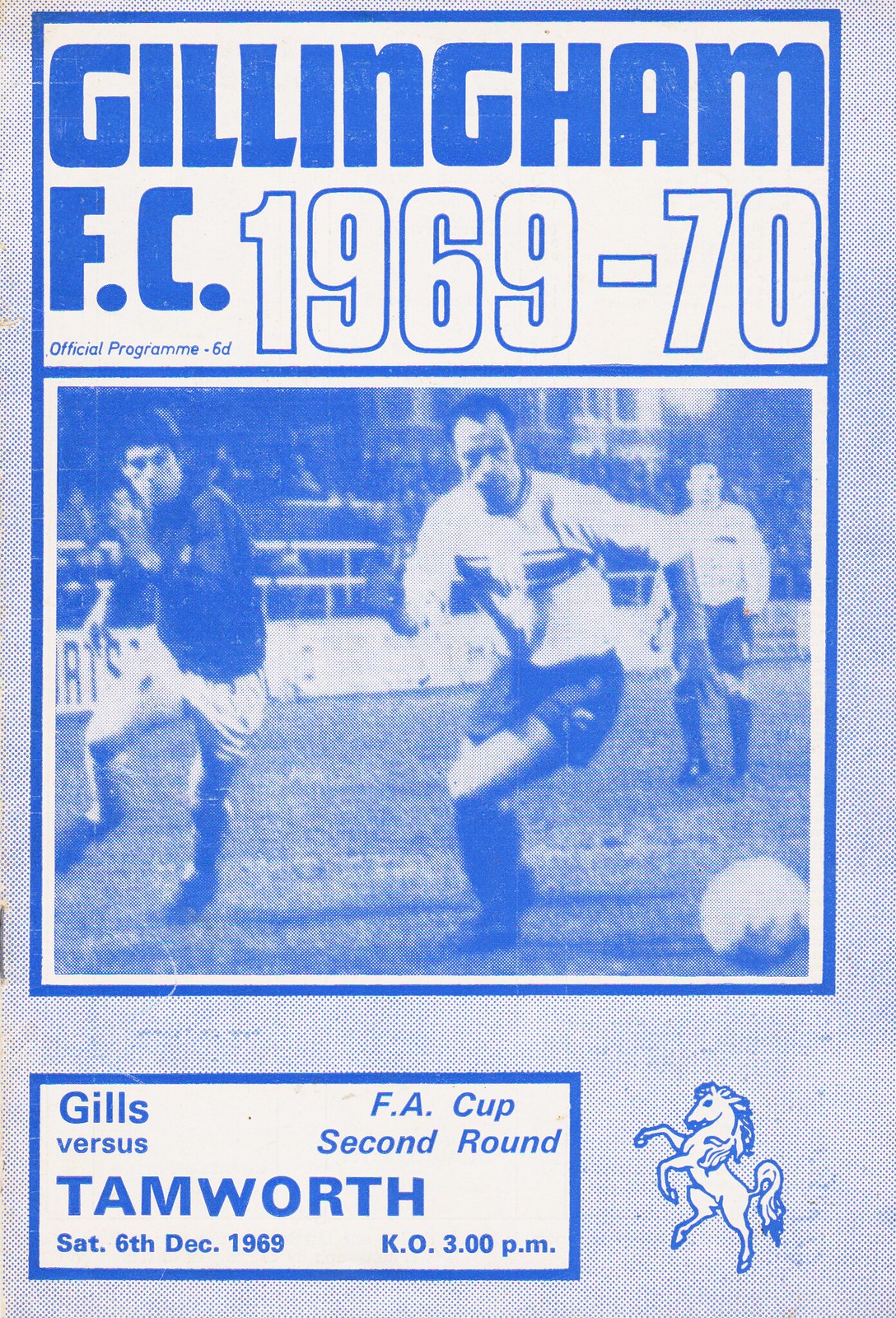This image is the cover of an official Gillingham FC soccer program from the 1969-70 season. The top of the cover features the headline "GILLINGHAM F.C." in large, bold uppercase blue font. Directly below, in larger white text with a blue border, it reads "1969-70" alongside the phrase "official program 6D." The center of the cover is dominated by a blue and white photograph of two footballers vying for the ball, one in a white shirt and the other in a dark shirt. The bottom part of the cover features a white rectangle with blue print detailing the match: "Gills vs. Tamworth, Saturday, 6th December 1969, kickoff 3:00 p.m." Additionally, it notes that this is the FA Cup second round matchup. The background of the frame has a light blue fabric-like texture. Completing the design, there is a rearing stallion logo situated in the lower right corner.